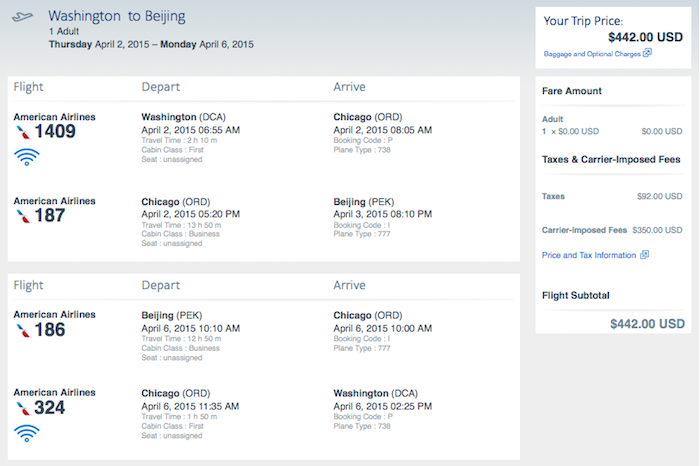This image depicts a flight booking page from a travel website. In the top left corner, there is a small airplane logo encased in a blue border with the text "Washington to Beijing" to its right. Below this, the details read "One Adult, Thursday, April 2, 2015 - Monday, April 6, 2015."

The main section of the page includes two boxes. The first box is divided into three columns labeled "Flight," "Depart," and "Arrive." Under "Flight," the itinerary lists "American Airlines 1409" and "American Airlines 187." The "Depart" column shows "Washington, DCA, April 2, 2015, 6:55 AM," followed by "Chicago, ORD, April 2, 2015, 5:20 PM." The "Arrive" column indicates "Chicago, ORD, April 2, 2015, 8:05 AM," and "Beijing, PEK, April 3, 2015, 8:10 PM."

In the top right corner of the image, the trip price is displayed as "$442 USD." Below, another box breaks down the fare amount: "Adult, 1 x $0," "Taxes and Carrier Imposed Fees," with "Taxes: $92" and "Carrier Imposed Fees: $350."